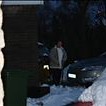A small, heavily cropped photograph depicts a person standing between two cars. The individual is dressed in a tan winter jacket over a white shirt. The ground is covered with a large amount of snow, with faint footprints visible. To the side, there's a partial view of a brick wall with a green trash can in front of it. One of the cars next to the person appears to be a sedan. In the background, trees are faintly discernible, contributing to the wintry atmosphere of the scene.